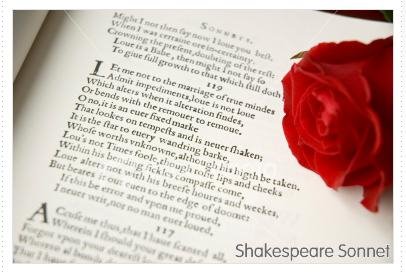This image captures a page from a book, specifically featuring one of Shakespeare's sonnets, which is indicated at the bottom of the page by the text "Shakespeare sonnet." The photograph is presented in landscape view and provides a detailed, artistic representation. On the right-hand side, there is a red rose laid delicately across the page, emphasizing the romantic theme often associated with Shakespeare's work. 

The sonnet begins with the partially legible line, "Might I not then lay now I love you less best." However, much of the text is intentionally blurred, focusing the viewer's attention on selected clear portions. Among the discernible lines, phrases like "Love it a babe, then might I not fay, foe," and snippets from Shakespeare’s iconic Sonnet 116, including "Love is not love which alters when alteration finds," are visible. 

The image is a close-up shot that captures the page slightly diagonally, adding to its artistic appeal. The book’s binding is slightly visible on the left-hand side, showing a glimpse of the adjoining page, while the upper right-hand corner features a small black triangle due to the angle of the shot. The sonnet is set against a stark white background with predominantly black text, varying in clarity and font darkness, thereby enhancing its visual complexity and artistic depth.